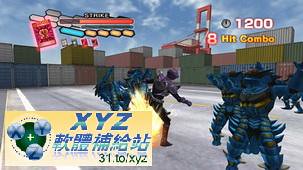This is a detailed caption for the image provided:

"This image captures gameplay from a video game featuring text possibly in Chinese, Japanese, Korean, or another similar script, possibly Mandarin. In the center of the screen, there are five or six characters adorned in body armor with scale-like or thorny details on the sides. The left-hand corner of the screen displays a gauge likely indicating the characters' remaining life. The top-left section features numbers showcasing what may be the characters' health points. On the right-hand side of the screen, text reads '21208 hit combo' in large, prominent font. Three of the armored figures are clustered together in the upper portion of the screen, while two others are positioned underneath them on the opposite side, forming a dynamic tableau suggesting intense action or combat."